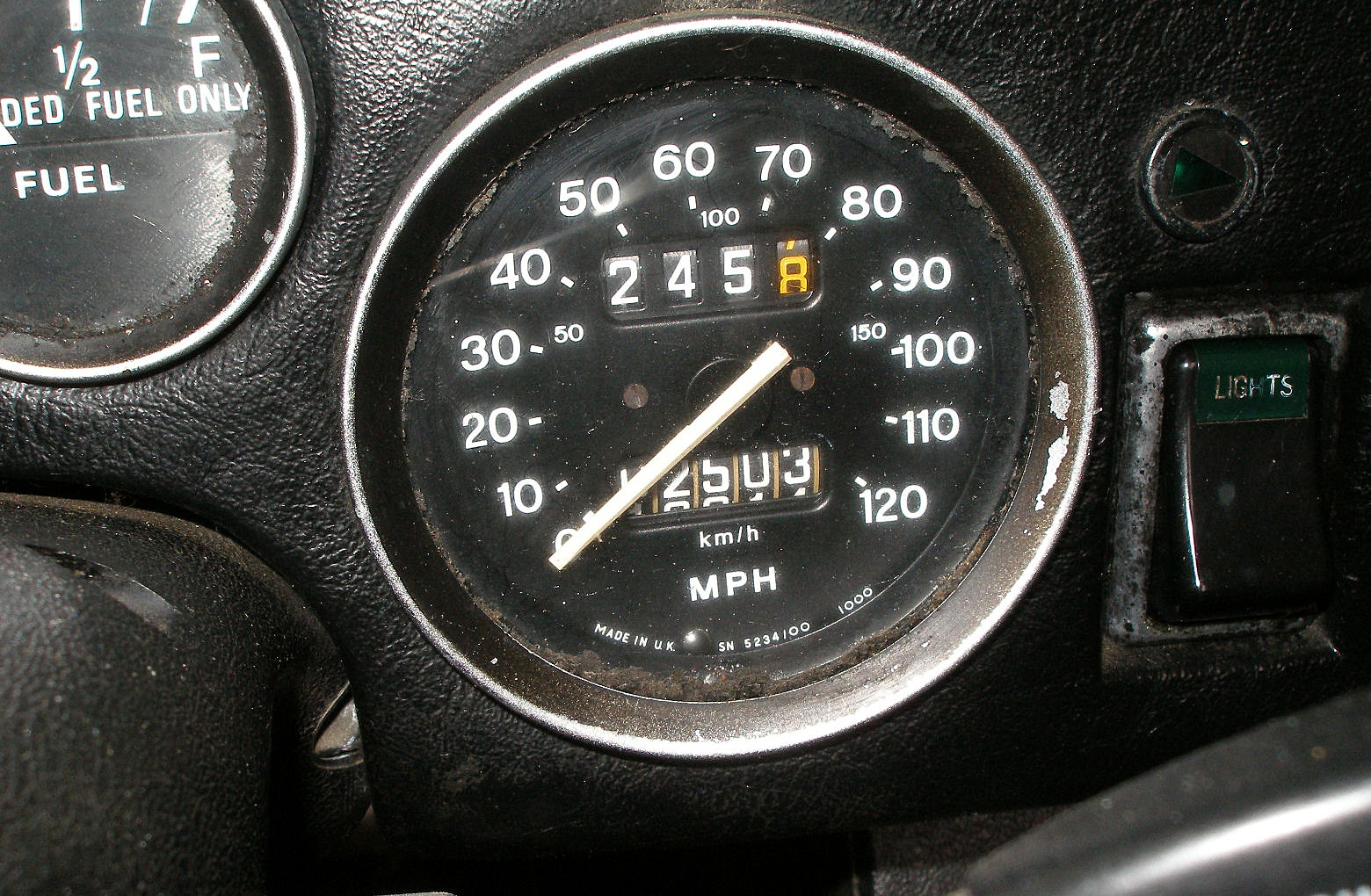This color photograph captures the intricately designed control panel of a vehicle, showcasing a luxurious black leather dashboard. Situated in the top left corner is the fuel gauge, partially obscured with text that reads "DED fuel only." The gauge displays marks for a half-tank and a full-tank, labeled "½" and "F," respectively, though the needle is not visible. Dominating the center of the image is a round speedometer with a white needle fixed at the zero mark. The speedometer features gradations ranging from 0 to 120, and at its top center, the odometer reads "245," with the digit "8" poised to change. The number "8" stands out in yellow against the rest. Below this is a smaller odometer, though partially cropped, revealing the numbers "2503" with additional text indicating "KM/H," "MPH," and "Made in UK," followed by the serial number "SN5234/001000." To the right side of the panel, a black light switch is visible, clearly marked with the word "Lights" in crisp white lettering.